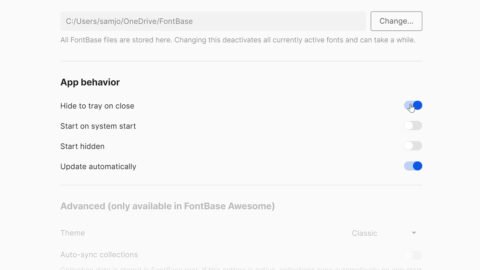Screenshot Description: Detailed Display of SamJoe OneDrive Font Base Settings

In this screenshot, the address bar prominently displays the text "See? Uses SamJoe OneDrive Font Base." To the right side of this bar, there is a clickable box labeled "Change." Beneath this section, there is informational text stating, "All font base tiles are stored here. Changing this deactivates currently active fonts and can take a while."

The section below this message is titled "App Behavior" in bold, black font. Directly beneath, there's an option labeled "Hide to Tray on Close," accompanied by a horizontal slider that can be toggled left or right. When slid to the right, the slider appears blue, indicating activation. Currently, "Hide to Tray on Close" is toggled on (blue).

Further down, there is a list of additional settings:
- "Start on System Start," which is not activated.
- "Start Hidden," also not activated.
- "Update Automatically," which is turned on.

Towards the bottom, there is a lighter, boxed section labeled "Advanced," indicating that this feature is only available in the Font Base Awesome version. Additionally, within this faint area, there are the words "Theme" and "Auto Sync Connections," visible but not prominently highlighted.